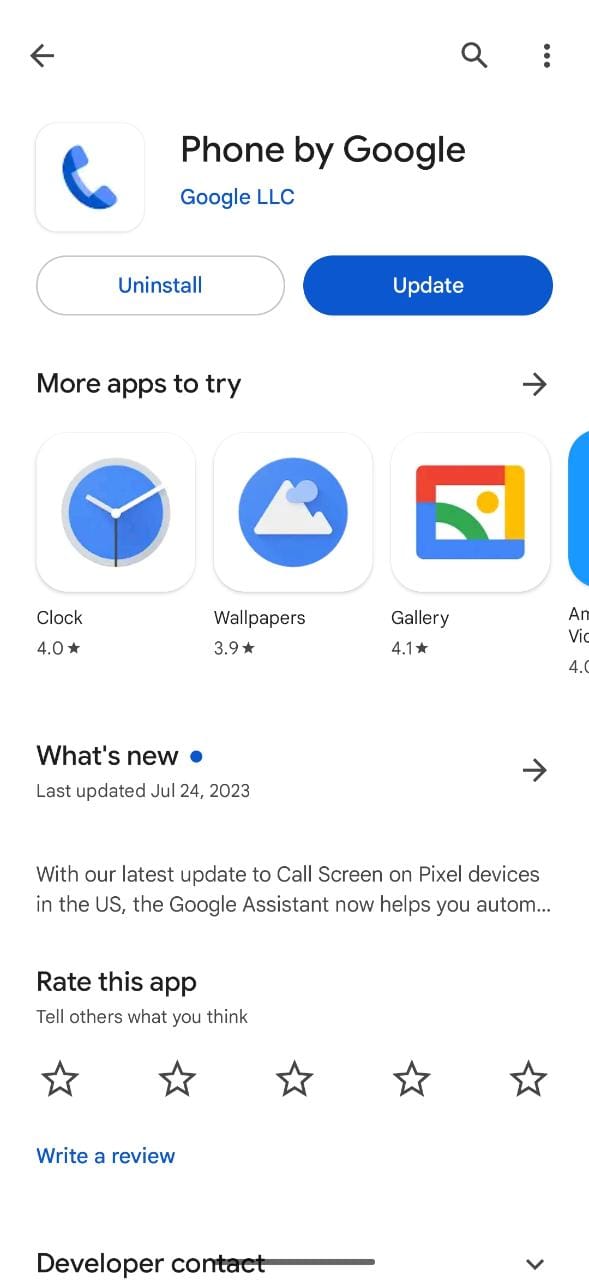This screenshot from the Google Play Store features the "Phone by Google, Google LLC" app. The app icon displays a blue phone receiver on a white background. The app name "Phone by Google, Google LLC" is prominently displayed at the top, accompanied by two primary action buttons: "Uninstall" on the left and "Update" on the right. 

Below the buttons, there's a "More Apps to Try" section showcasing icons for additional apps like Clock, Wallpapers, and Gallery, though some app icons are not fully visible. Moving further down, a "What's New" section highlights the latest update dated July 24th, 2023, noting enhancements to the Call Screen feature on Pixel devices in the US, powered by Google Assistant.

Beneath the update details, there is a "Rate This App" section with an option to rate the app out of five stars, along with a link to write a review. Partially visible at the bottom of the screenshot is the developer's contact information, though the specifics are obscured.

In summary, the screenshot illustrates how users can update or uninstall the Phone by Google app, provides a brief glimpse of related apps to explore, and outlines the most recent feature improvements as of July 24th, 2023, with more detailed update information accessible upon further interaction.